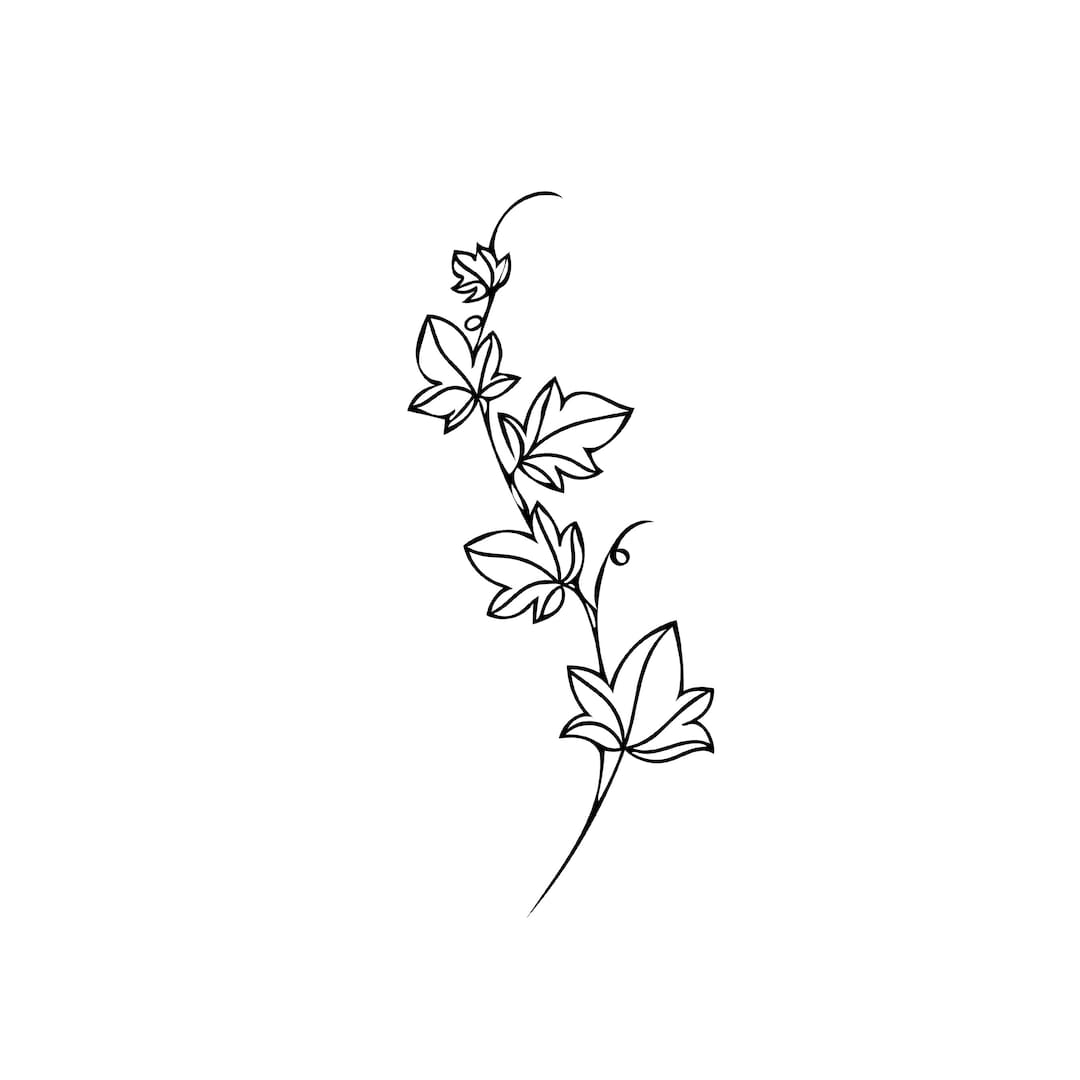The image depicts a simple, black ink illustration of a slender, curved stem set against a white background. The stem, which starts at the bottom middle and extends to the central top, bears five leaves arranged in an alternating pattern. The first leaf, positioned at the bottom right, has five distinctive veins conjoining at its base and spreading out towards the edges. Ascending the stem, the second leaf appears on the left side, followed by the third on the right, the fourth on the left, and the fifth, significantly smaller, near the top center. All leaves share a similar structure with five pronounced points: two on either side and one larger central point. Each leaf's veins are meticulously drawn, emphasizing the detailed, sketch-like nature of the artwork.